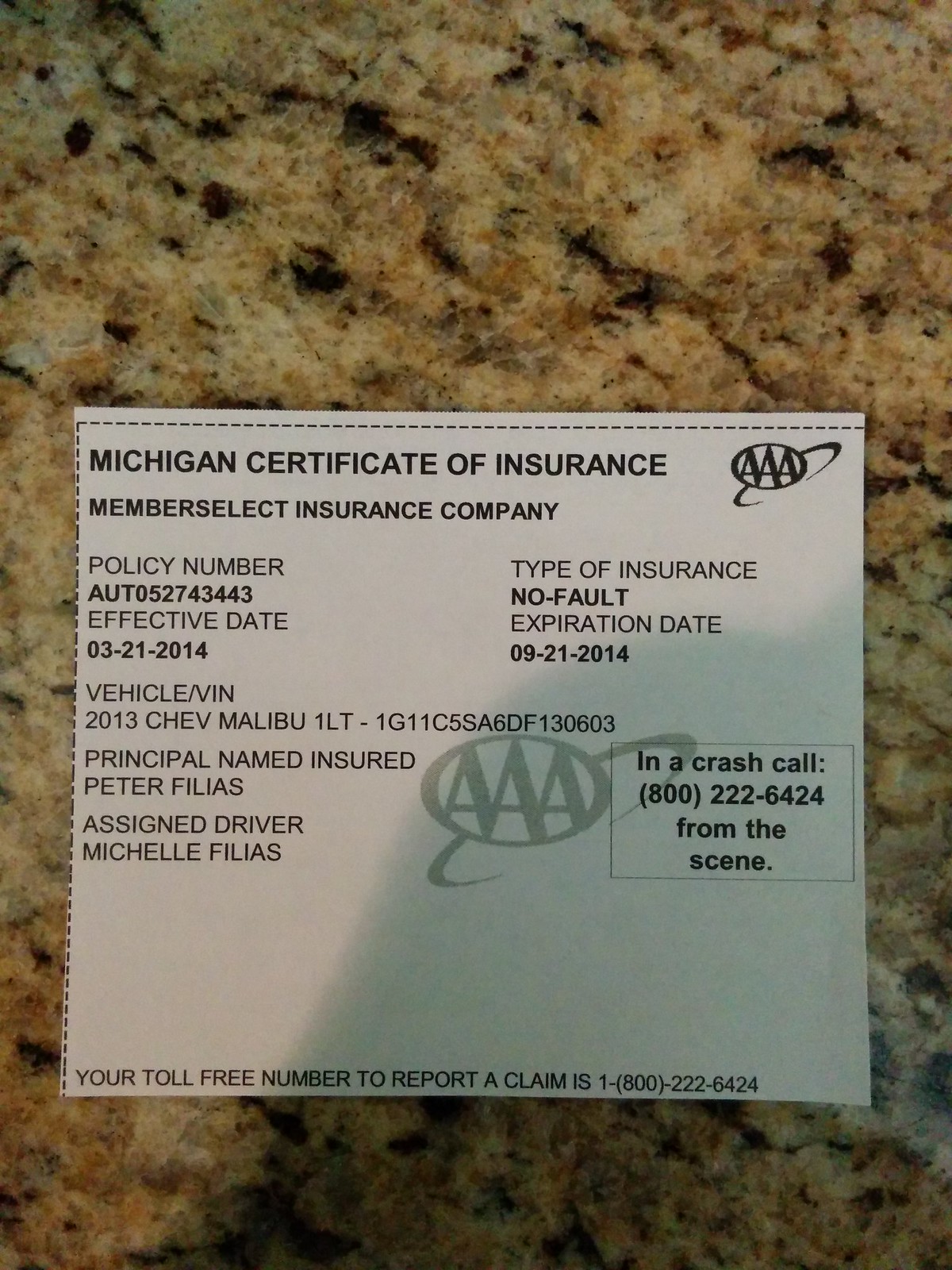The vertically aligned rectangular picture features a brown and black speckled granite countertop. Centered on the countertop is a white, square-cut piece of paper, labeled "Michigan Certificate of Insurance" in all caps black letters at the top, followed by "Member Select Insurance Company." On the upper right-hand side, an AAA logo can be seen, with another AAA logo serving as a faint watermark in the center of the paper. The text is primarily left-aligned and provides the following details: 

- Policy Number: AU2052743443
- Effective Date: 03-21-2014
- Expiration Date: 09-21-2014
- Type of Insurance: No Fault
- Vehicle VIN: 1G11C5SA6DF130603 for a 2013 Chevy Malibu 1LT
- Principal Named Insured: Peter Fillius
- Assigned Driver: Michelle Fillius

Additionally, a small box on the right side of the paper advises, "In a crash call 800-222-6424 from the scene." At the bottom, it also provides the information "Your toll-free number to report a claim is 1-800-222-6424."